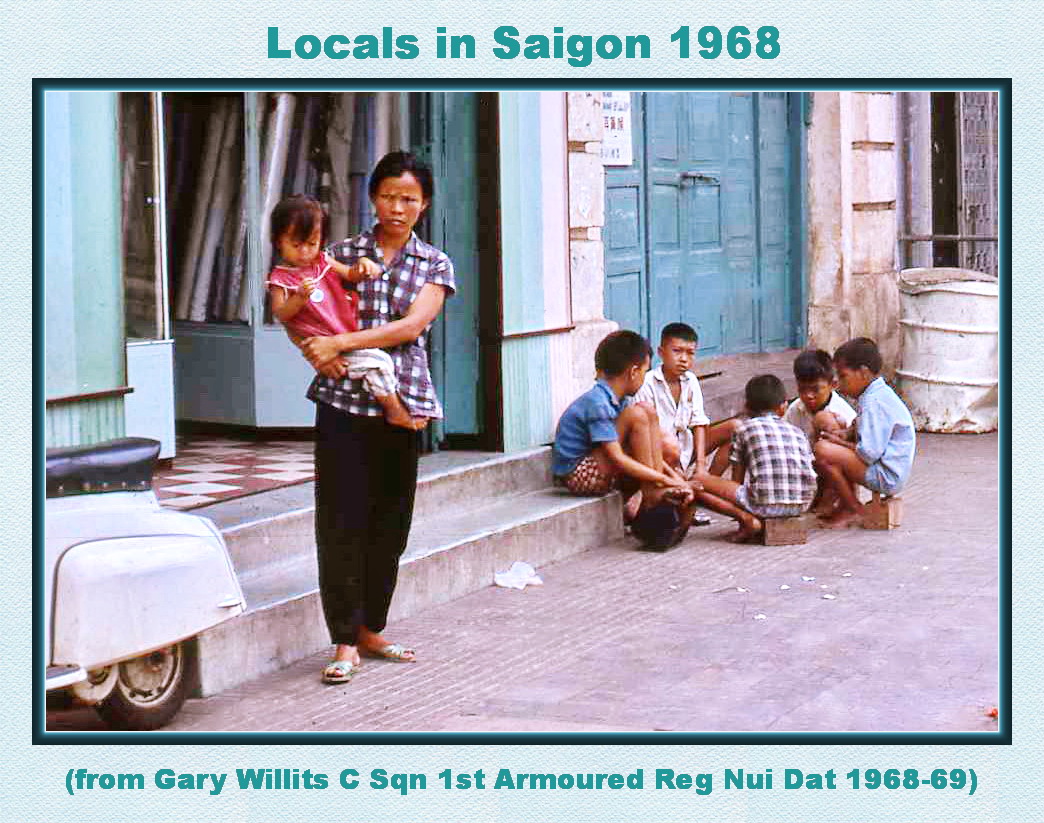This image, framed within a light blue cardstock border that reads "Locals in Saigon, 1968" at the top and "From Gary Willett, C-Squadron, 1st Armored Regiment, Nui Dat, 1968-69" at the bottom, captures a poignant scene in a poor-looking area during the daytime. The photograph, rectangular and slightly grainy, shows a street lined with shops or open buildings on the left. In the lower left-hand corner, the back end of an older-looking scooter is visible. 

Center stage is a woman with a sullen expression, standing in the doorway of a business or house. She is holding a baby dressed in pink, while she herself wears a checkered button-up shirt and black pants. Behind her are concrete steps leading up to her building, flanked by a set of blue doors. 

To her right, a group of children, dirty and barefoot, are sitting in a circle on the sidewalk and small boxes, engaged in a game. Amongst them is a beat-up drum lying on the street. The overall scene, rich in detail yet somber, encapsulates a moment of daily life amidst the backdrop of Saigon during 1968.